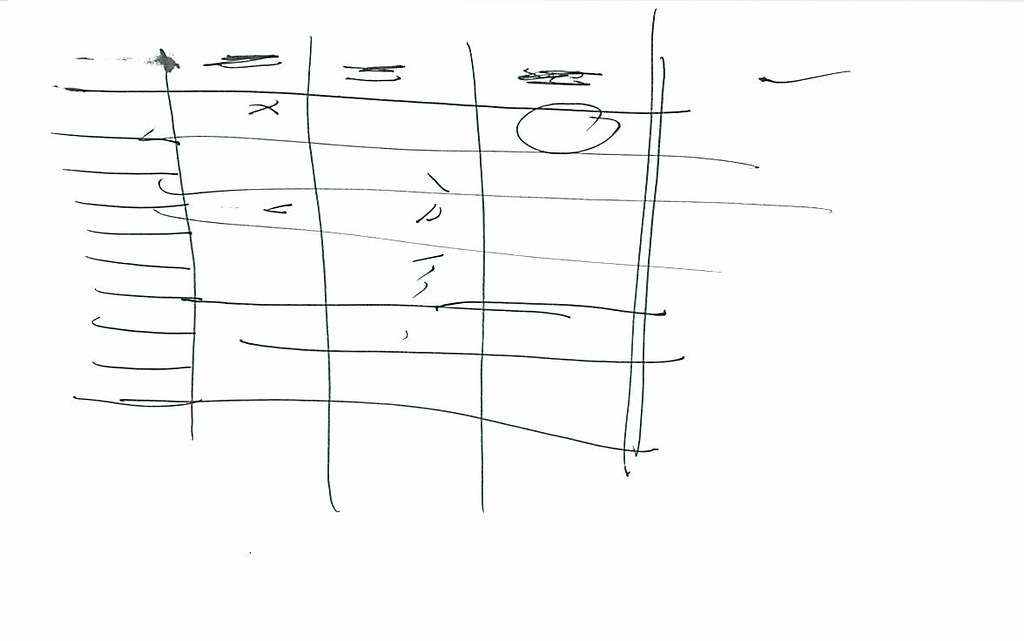The image is a scanned white paper featuring a human-drawn grid with black ink. The grid has 7 rows and 4 columns, with variations in the number of dividing lines within each column. The first column contains 10 horizontal dividing lines, while the other three columns each have 7. 

At the top of the page, there are faint scribbles that appear to obscure something, but no discernible text or numbers are visible beneath. Specific markings within the grid include:

- An "X" in the cell at row 2, column 2.
- Scribbles in the cells at row 4, column 2, and rows 3, 4, 5, and 6 of column 3.
- A neatly drawn circle in the cell at row 1, column 4.

No alphanumeric characters are present; the image only contains these various shapes and markings.